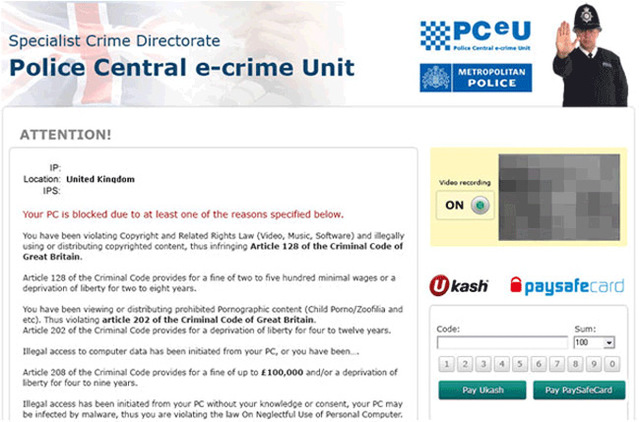In this image, the upper left-hand corner features a graphic of the British flag, overlaid with the text "Specialist Crime Directorate, Police Central E-Crime Unit." Adjacent to this, in the upper right corner, the text reads "PCEU," with "Police Central E-Crime Unit" right below it. Below this text, within a blue box, are the words "Metropolitan Police." Embedded in this section is an image of a British officer adorned in a distinctive hat, extending a hand toward the camera with the palm open.

To the right side of the page, beneath this box, text in red declares "Video Recording On," alongside a green indicator button and a rectangle displaying a blurred gray area. Below this text, it reads "U-Cash," accompanied by an image of a padlock and the label "Pay Safe Card." The section prompts for a code entry with an empty text box labeled "SUM 100," followed by a numeric keypad displaying numbers 1 through 9, with a zero at the end. The options "Pay U-Cash" and "Pay Safe Card" are also available.

The left side of the page states "IP Location, United Kingdom," and continues with an alert: "Your PC is blocked due to at least one of the reasons specified below." It accuses the user of violating copyright laws by illegally using or distributing copyrighted content, infringing Article 128 of the Criminal Code of Great Britain, and enumerates the associated criminal penalties. It further accuses the user of viewing or distributing prohibited pornographic content, citing specific article numbers and penalties. Additionally, it claims that illegal access to computer data has been initiated from the PC, possibly without the user’s knowledge or consent, indicating that the PC may be infected by malware and thus violating the law on neglectful use of a personal computer.